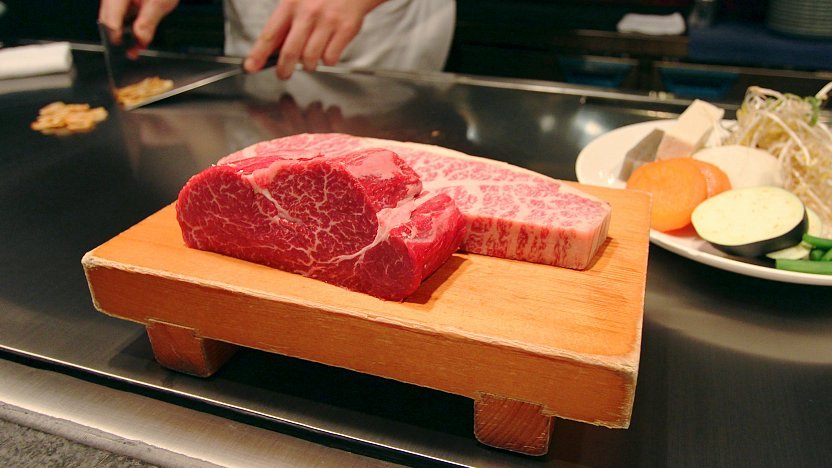In the bustling scene of a teppanyaki restaurant, a skilled chef, visible from the hands donning an apron, attends to a sizzling grill in the back left. The focus is on a small wooden butcher block in the foreground, displaying two marble-rich cuts of meat, a filet mignon and what appears to be either a New York strip or a ribeye, likely high-grade Japanese Wagyu A5. To the right of the meat-laden block, a plate garnished with a vibrant assortment of sliced vegetables—carrots, tofu, beans, sprouts, and eggplants—catches some of the light, reflecting against the gleaming steel surface beneath it. The chef, dual-wielding spatulas, tends to some garlic chips on the grill, orchestrating a meticulous and visually appealing culinary experience in this clean, well-organized Japanese barbecue setting.